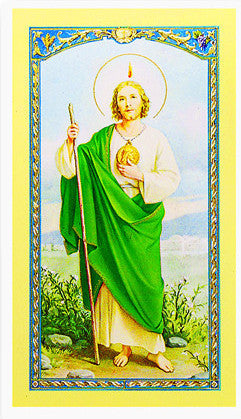This is a detailed depiction of a holy or prayer card featuring Christ. The card has an outer yellow border with an ornate blue and gold filigree design just inside it. At the center of the card is an image of Christ standing barefoot on the ground, flanked by bushes and rocks, with a mountainous landscape and what appears to be water directly behind him. 

Christ is depicted with medium-length blonde hair and is dressed in a white robe with a green robe draped over his right shoulder, covering his right bicep, and extending downwards. Around his neck hangs a large gold medallion that reaches towards his waist. In his right hand, he holds a long staff, further symbolizing his role as a shepherd and guide. 

Above his head is a red flame and a flaming circle, symbolizing holiness and divinity. The overall composition and details point to this being a religious image, likely used for prayer or reflection.